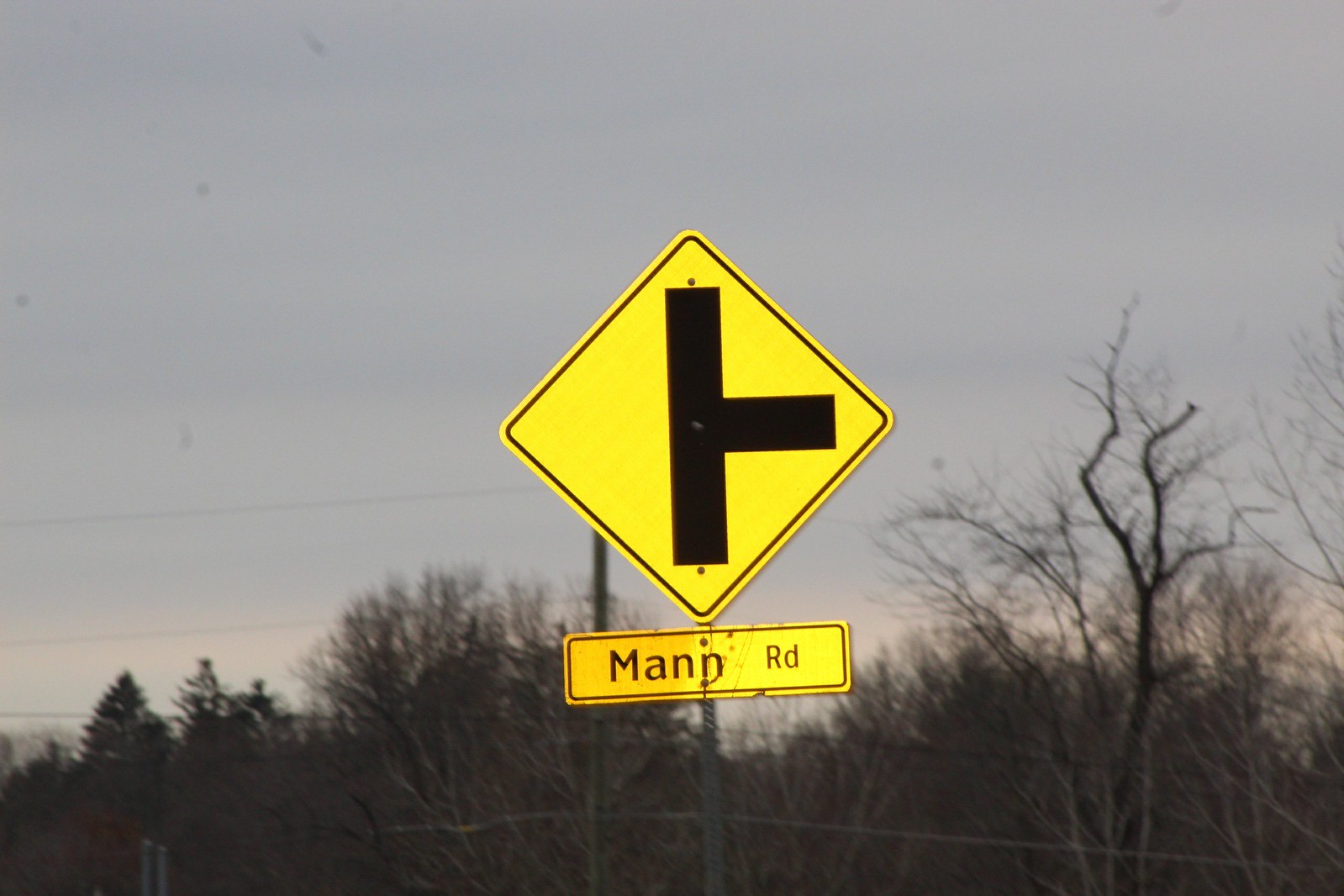The photograph captures a street sign at dusk. The sky is transitioning into evening, adorned with a gradient of deep blue and soft purple hues. The horizon retains a subtle brightness, offering the last glow of daylight. In the background, barren trees on the right side suggest the chill of fall or winter, while a trio of pine trees on the left adds contrasting greenery.

Dominating the foreground is a distinct yellow street sign, shaped like a diamond but oriented with a point upward and another downward. The sign features a bold, black vertical line intersected by a shorter black line branching off to the right, indicating an impending intersection on the right side of the road. Encircling the yellow portion is a black border, providing clear visibility. Below the main sign, a smaller rectangular sign displays the text "MANN RD" in all capital letters, designating the street's name.